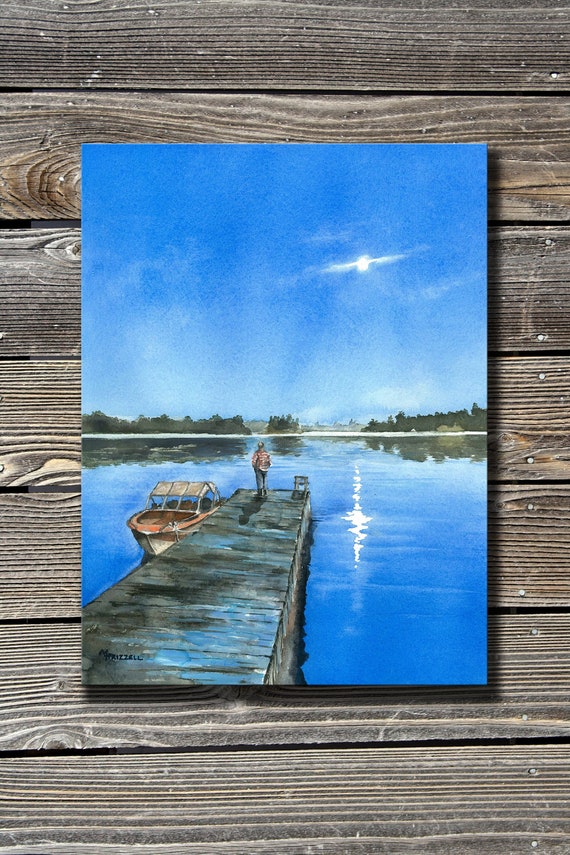The detailed image depicts a painting set against the backdrop of a wooden surface, which appears to be an outdoor table characterized by its grayish-brown color and comprised of seven horizontal planks, each with distinct grain patterns and visible knots. The planks are held together by nails, and there are black gaps between them. Within this setting, the painting itself forms a smaller, portrait-oriented rectangle.

The painting portrays a serene scene of a pier extending from the lower left and heading towards the center of the image. The pier is depicted in shades of brownish-gray with touches of light blue, presumably due to the effect of sunlight. At the end of the pier stands a person, dressed in a reddish-brown jacket and dark blue jeans, gazing out across a vibrant blue sea. 

To the left of the pier is a small boat, likely motorized, with its nose pointing towards the land and its stern facing the open water. The boat's interior is muted red while the exterior is white, featuring a small roofed section over the seating area.

The body of water, which looks like a lake, is a rich blue that lightens closer to the foreground, reflecting the sun and sky in its surface. The sun is positioned slightly to the right of the center in the sky, almost resembling the rings of Saturn. The horizon line bisects the painting horizontally, with a low row of trees on both the left and right sides, creating a mirrored image on the water. The sky transitions from a cloudy white at the bottom to a medium blue at the top, harmonizing with the similarly blue water below.